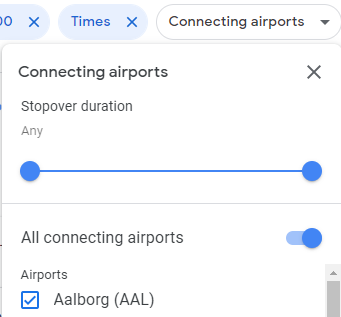The screenshot showcases the top-right corner of an app or website interface for booking flights. At the top, several options are available, although only the "Times" option is fully visible. "Times" is highlighted in a slightly oval, blue-outlined box with the word "Times" in blue text and a blue 'X' to its right. To the left, there's another partially visible option, showing only an "O" and a blue 'X'.

Below these options, there is a similar shaped white box labeled "Connecting Airports," which features a dropdown menu. The title "Connecting Airports" is followed by the label "Stopover Duration," next to which there is an "Any" option and a slider bar. This slider presumably allows users to select any airport for the stopover duration or adjust it to choose airports with shorter stopovers.

A separator line divides this section from the subsection titled "All Connecting Airports," adjacent to which there is a blue slider switch set to the "on" position. Below this, a list begins, displaying "Airports" as the header, with the first item in the list being "AALBORG," marked by a tick in a checkbox. To the right, part of a menu bar is visible, indicating more content relevant to selecting airport connections.